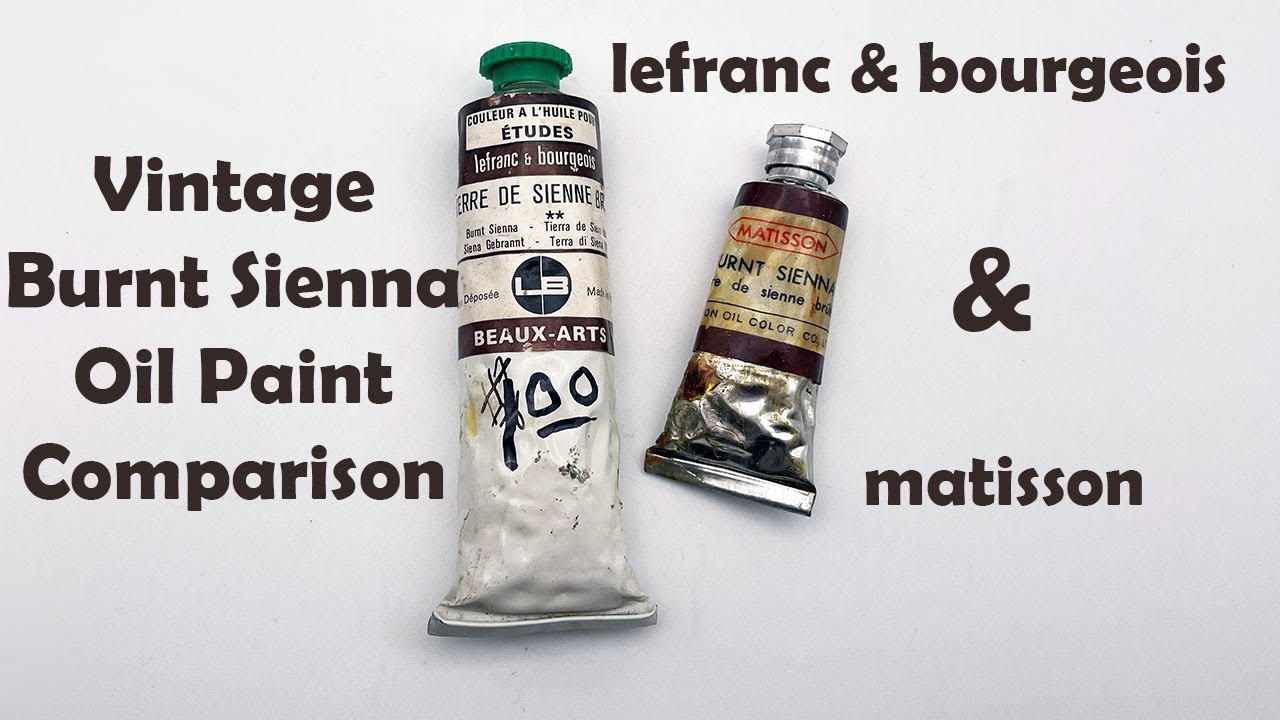The image features two vintage oil paint tubes set against a neutral background, aligned vertically but slightly angled away from each other at their caps. The larger tube, positioned on the left, has a green cap and a predominantly white metal body adorned with brown labeling. This tube is identified by text reading "Vintage Burnt Sienna Oil Paint Comparison" along its side. The smaller tube on the right, approximately half the size of the left tube, has a silver cap and a mostly silver body, likewise decorated with brown and yellow labeling. The label on the right tube prominently features the text "LaFranc & Bourjois" followed by "Matisson." Both tubes exude a nostalgic, vintage aesthetic reminiscent of old metal toothpaste containers.